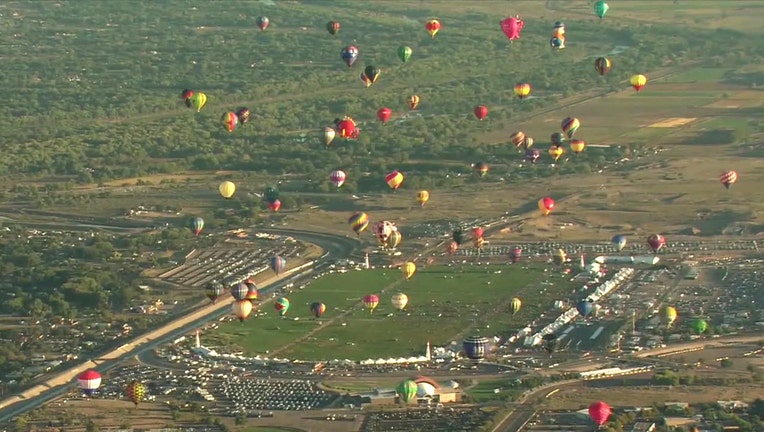In this breathtaking aerial photograph, dozens, if not hundreds, of vibrant hot air balloons of various shapes and colors fill the sky, creating a spectacular display. The perspective suggests the image might have been captured from another hot air balloon, an airplane, or a drone. Below, a large, open field, possibly a football or track field, serves as the launch site, surrounded by numerous parked cars in an adjacent parking lot. A freeway snakes from the bottom left corner, adding a dynamic element to the scene. The landscape is richly detailed with lush green forests on the left and neatly plowed farmland on the far right. Scattered houses and outbuildings dot the terrain, adding a human touch to this picturesque setting. Altogether, this image vividly captures the joyous and colorful spectacle of a hot air balloon festival set against a beautifully varied landscape.